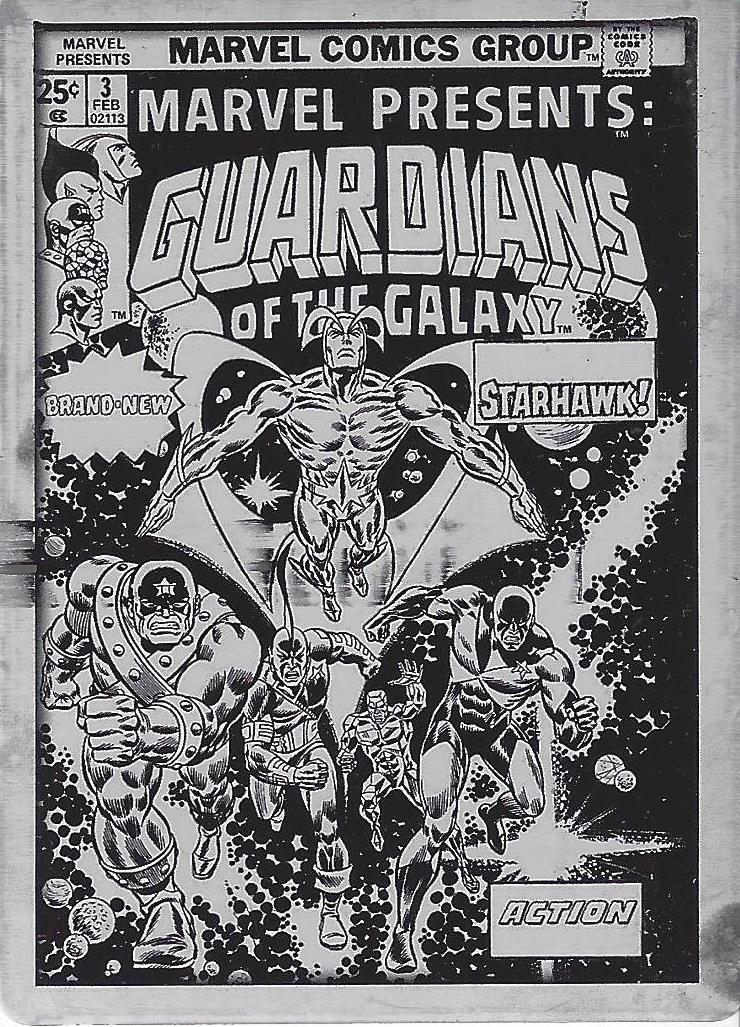This image depicts a black and white recreation of the front cover of a Marvel comic book, specifically the number three issue of "Guardians of the Galaxy". At the very top, in black text, it reads "MARVEL COMICS GROUP" in all capital letters. Below this, "Marvel Presents" is mentioned twice, once on the left side and again in white text against a black background. To the left, the price is displayed as 25 cents, along with the date "3 February, 02113". The title "Guardians of the Galaxy" is prominently featured with a 3D effect. The cover also promotes "Brand New Starhawk Action". The imagery includes various characters with angry or determined expressions; Starhawk is depicted flying towards the viewer, while other characters appear to be running. Notably, familiar characters such as the Silver Surfer are also present.